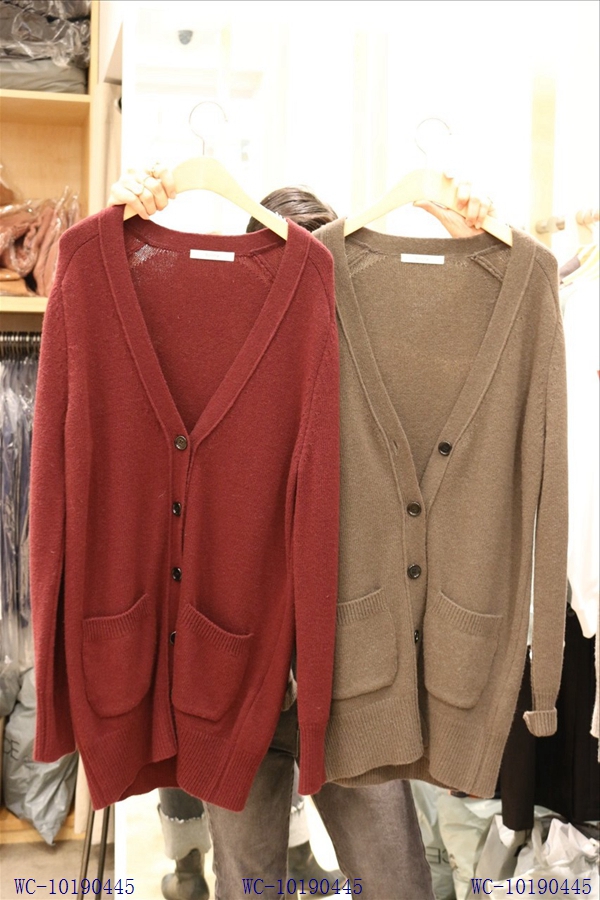In a store setting, a person with dark brown hair, partially obscured by the sweaters they hold up, showcases two v-neck cardigan sweaters on wooden hangers. The person's jeans are barely visible beneath the hem of the sweaters. The sweater on the left is maroon or dark red with black buttons, featuring a top button that is fastened and two front pockets. The sweater on the right is an olive green, also with black buttons, but its top button is unfastened. Both cardigans hang open, revealing their classic style. In the background, shelves display additional merchandise, including clothing in plastic bags and other garments on hangers. The area is marked with some watermarks labeled WC-101-90445.